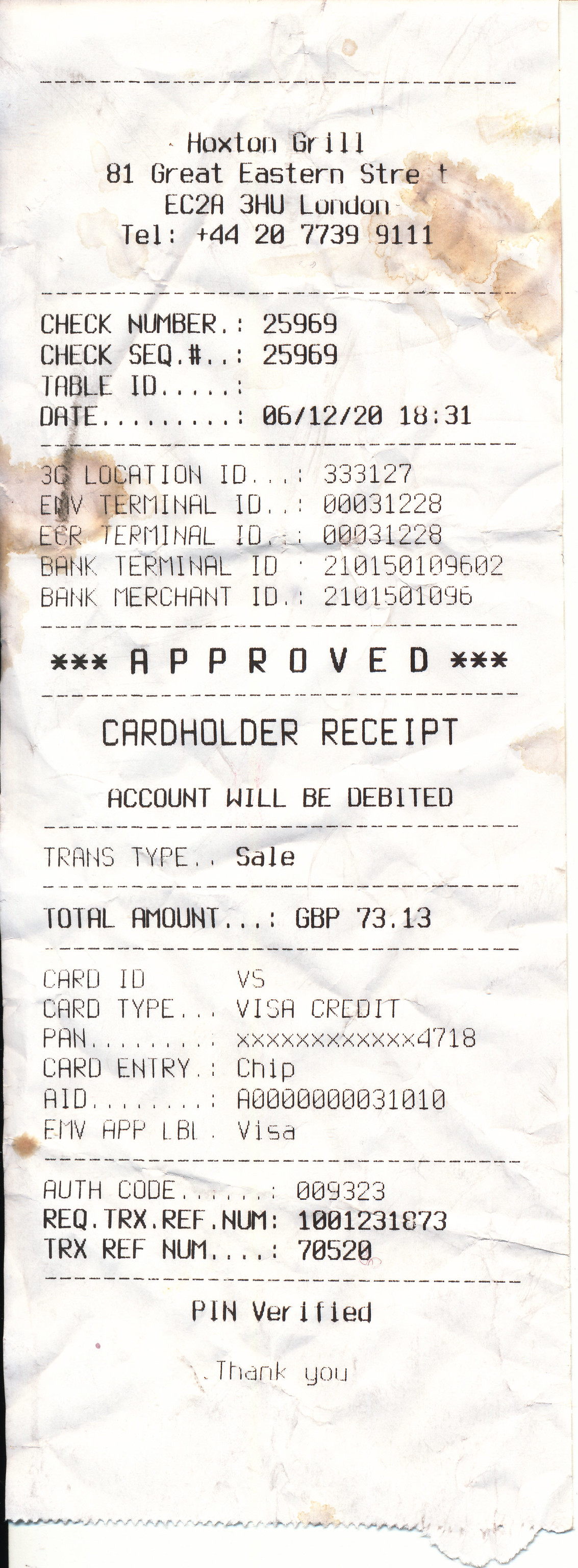This image depicts a worn and slightly crumpled cardholder receipt from Hoxton Grill, located at 81 Great Eastern Street, London, EC2A 3HU. There is noticeable staining, which may be brown streaks or possibly blood, across the upper and middle sections of the white paper. The receipt starts with the establishment's details, followed by a check number and check sequence both labeled 25969. It also includes a blank field for the table ID, and a date and time listed as 06-12-20 10:31. Below this section, various terminal and location IDs are provided. Prominently, the word "Approved" is printed horizontally with asterisks on either side, followed by a larger text reading "cardholder receipt". The receipt confirms the account will be debited, lists the transaction type as a sale, and shows a total amount of GBT 73.13. Further details include credit card information, authorization numbers, and a statement verifying the PIN. The receipt concludes with a small notation saying "thank you" at the bottom.